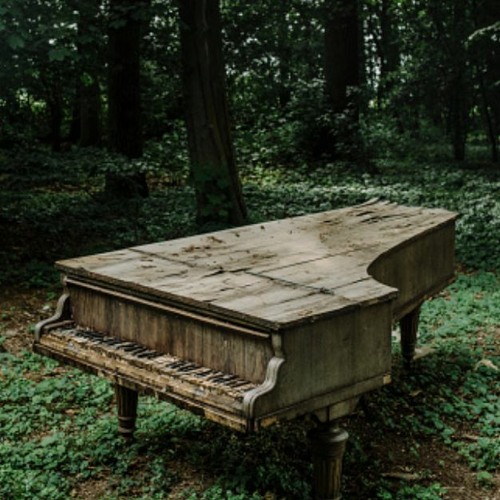In the heart of a dense, towering forest, where the trees form a thick canopy allowing minimal light to penetrate, stands an abandoned piano. This rustic, weather-beaten instrument, constructed entirely of wood, has clearly seen better days. It sits on a clearing with moss and clovers slowly creeping over its ornate legs, which remain somewhat less worn than the rest of the structure. The piano's layered top and wood panels are heavily decayed, with significant peeling and warping from prolonged exposure to the elements. Its keys, now warped and discolored, bear the marks of time, weather, and likely various small creatures. Despite its dilapidated state, the piano retains a certain far-off elegance, set against a backdrop where the tree trunks form a tight-knit labyrinth, receding into a leafy jumble that obscures any glimpse of the sky. This highly detailed and scenic image captures a poignant juxtaposition of fading grandeur against the relentless and renewing forces of nature.